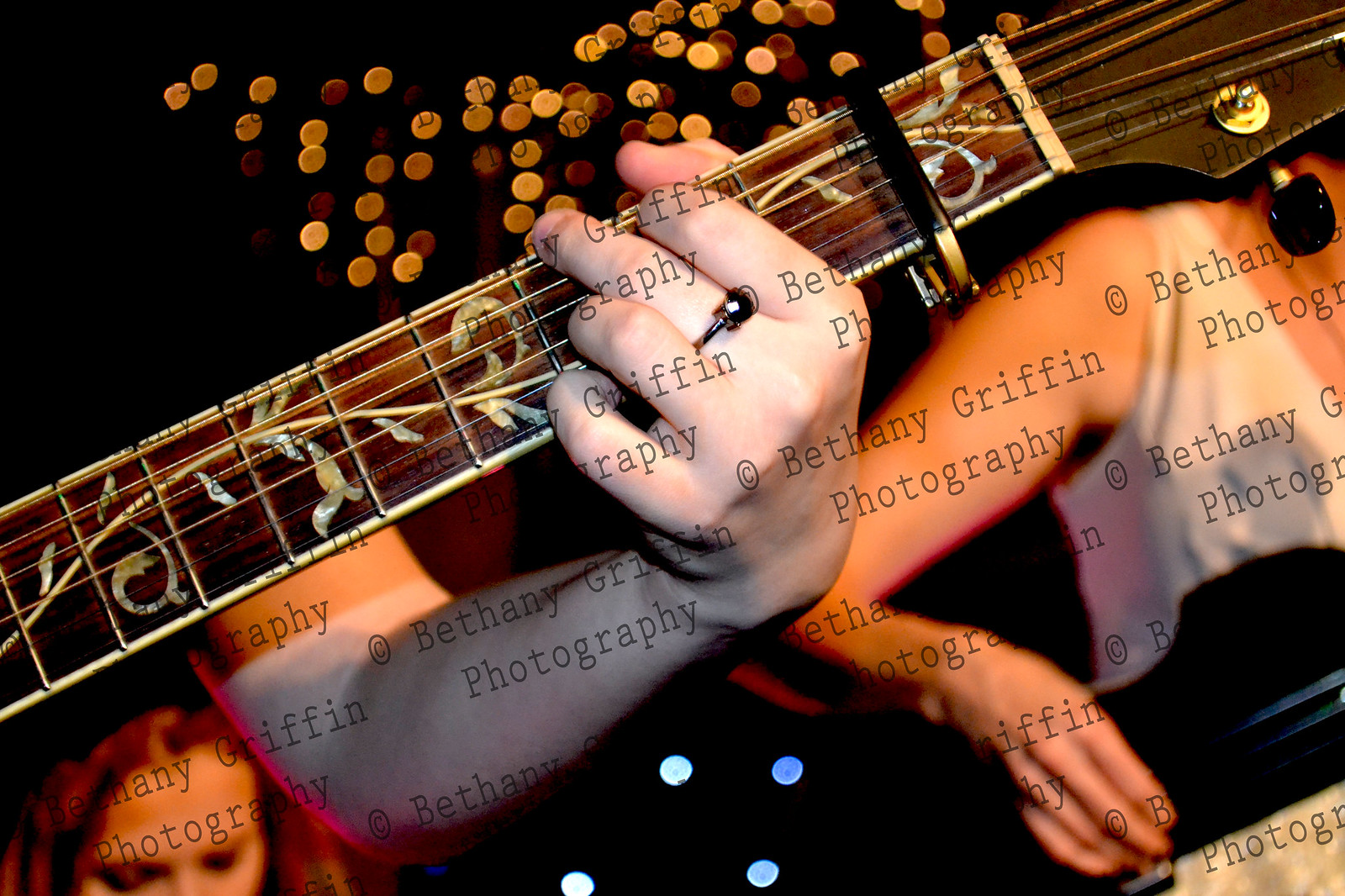This landscape-oriented photograph captures a close-up of a guitar’s fretboard, which features a decorative, iridescent shell inlay resembling a vine running the length of the neck. The focal point is a Caucasian left hand, possibly male, strumming the strings, adorned with a ring on the middle finger. To the right, partially visible, is another person wearing a white tank top, suggesting a second musician. The lower left corner of the image shows the top of a person’s head, revealing a forehead, eyes, and partially obscured nose, likely female. The background is intentionally blurred, with bokeh effects of gold, orange, and blue circular lights adding depth. The photograph is watermarked with "Bethany Griffin Photography."